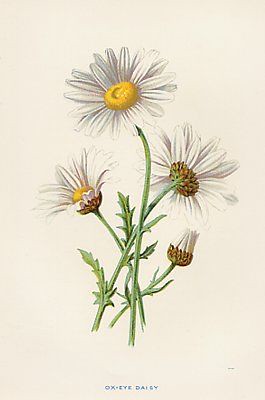This image is a detailed illustration of an Ox-eye Daisy plant, capturing four different stages of the daisy's evolution. At the bottom right, a daisy bud is fully closed, while to its left, slightly higher, a second bud is halfway open. The third daisy, positioned higher up on the right, is fully bloomed but faces away from the viewer, displaying only its back. The topmost daisy faces the viewer, showcasing its white petals and yellow center. All daisies have yellow centers, although not all are visible from every angle depicted. The daisy stems are thin and green, adorned with thorny, jagged-edged leaves, and appear slightly bent. The background of the illustration is off-white or yellowish, adding a vintage feel. This artistic rendition, possibly created with crayon or watercolor, is reminiscent of an encyclopedia or book page. Below the illustration, in small blue font, is the caption "Ox-eye Daisy."